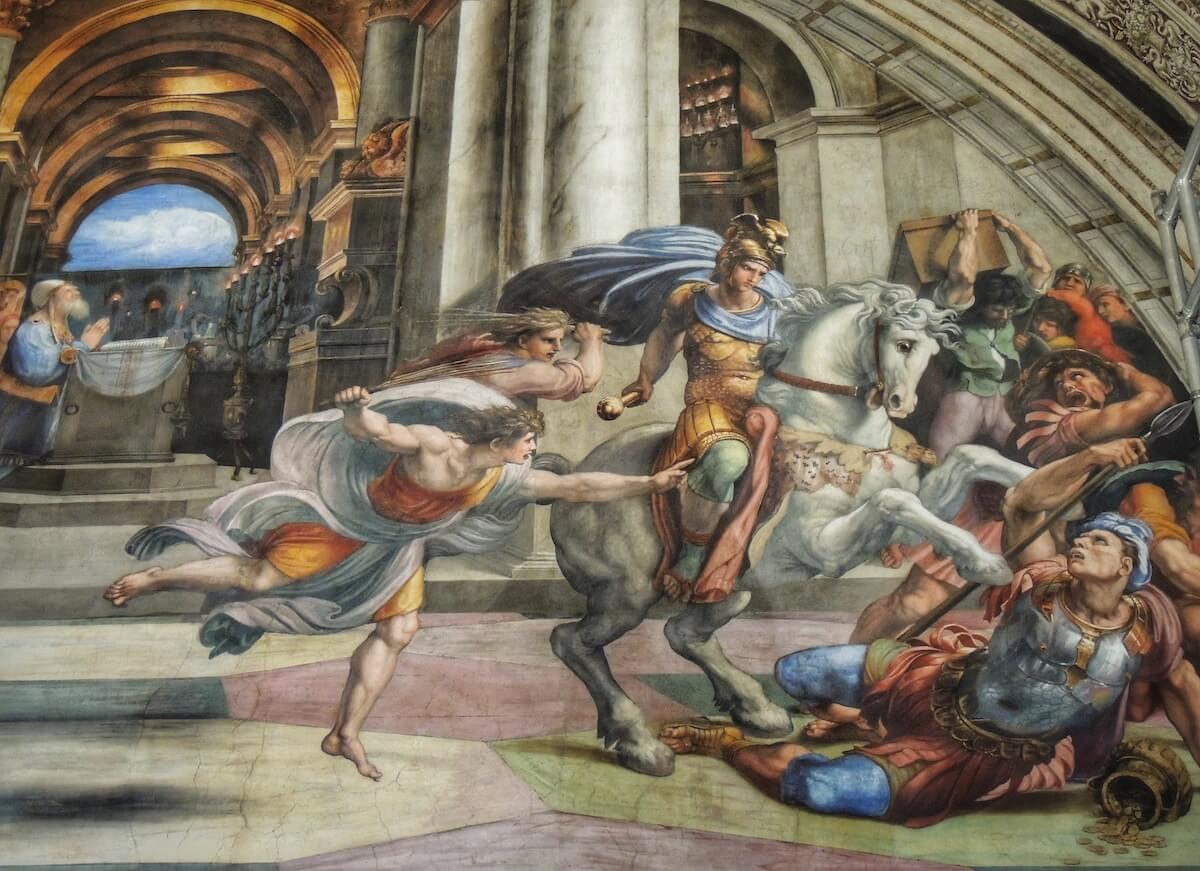This detailed painting depicts a chaotic Roman battle scene set in a lavish, ornate, large hallway or coliseum. The floor is a mosaic of multiple colors, and enormous marble columns line the space. The background shows a sprawling blue sky with clouds, visible through an expansive dome. Numerous figures are engaged in a frenzy of motion, depicted with a striking palette of red, orange, yellow, gold, blue, burgundy, white, gray, beige, brown, black, and pink hues.

Central to the scene is a Roman soldier, armored in gold with a blue cape and a golden helmet, mounted on a magnificent white horse. The horse, dynamic and powerful, appears to be trampling a fallen figure who lies in pain, clutching a spear beside a shattered vase spilling coins. Nearby, figures in desperate postures, including one praying figure, add to the scene's urgency and drama. To the right, additional combatants clash, some wearing blue pants and red smocks, while others in white smocks run and gesture.

The entire composition, almost square in its horizontal arrangement, captures the tumultuous and violent atmosphere of ancient warfare, with a blend of architectural grandeur and human struggle. The painting is rich in narrative and detail, conveying a vivid historical reenactment that is both dramatic and evocative.